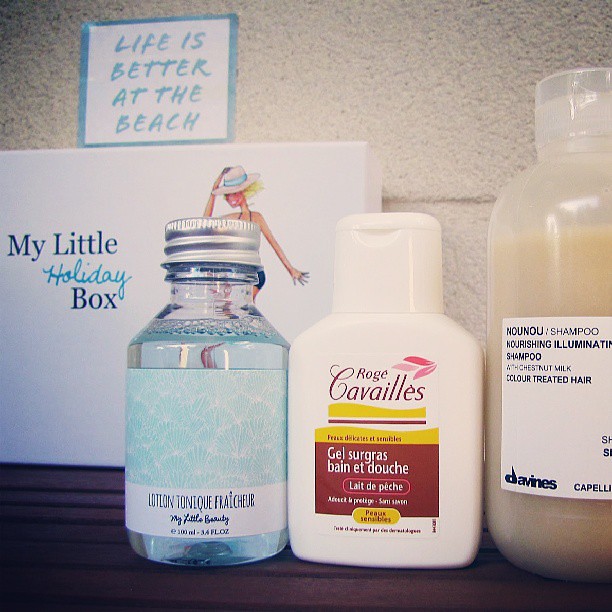This photograph features three distinct beauty products arranged side by side on a dark wooden table against a white, seemingly painted brick wall. At the center rear of the image, a white box with the inscription "My Little Holiday Box" in blue letters stands prominently. The word "holiday" is presented in a lighter blue and cursive script. Above this box, a small white sign with light blue text declares, "Life is better at the beach."

From left to right:
1. The first bottle is a transparent container with a silver screw-on cap and contains a clear liquid. The label reads "Lotion Tonique Fresh Air" and "My Little Beauty" in dark blue font, with additional small text detailing the volume of the product.
2. The middle bottle is white, resembling a squirt bottle, and bears the label "Roge Cavailes Gel Surgras." This label is marked by a red square with white text, along with additional white text in smaller fonts.
3. The bottle on the far right is partially cropped out of the image. It is a clear plastic bottle filled with a brown liquid, identified as a "nourishing shampoo" with chestnut milk, suitable for color-treated hair. The label includes the brand name "Davines" in lowercase black letters positioned at the bottom left.

The "My Little Holiday Box" features a charming, cartoon-like drawing of a woman dressed in a blue bikini and a white hat with a light blue band, partially obscured by the first bottle.